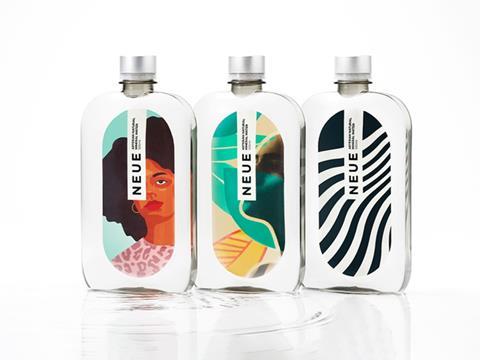This product image showcases three rectangular, flat bottles of a fragrance from the brand "Neue," spelled N-E-U-E, which means "new" in German. Each bottle, about a quarter of an inch thick, features a unique digital painting in the style of a watercolor. The leftmost bottle depicts an African-American woman with natural hair, wearing a light pink leopard print shirt against a teal background, looking slightly to the left. The middle bottle showcases an abstract design of a teal silhouette in front of teal and yellow leaves. The rightmost bottle is adorned with a black and white wavy stripe pattern, creating an abstract visual. All three bottles are capped with silver, screw-on caps and contain a clear liquid inside. They are set against a stark white background, appearing to be placed in a disturbed puddle of clear liquid, giving the image a clean and modern look. The central feature of each label is a white rectangle with the brand name "Neue" in black font, followed by three lines of text next to the "E."